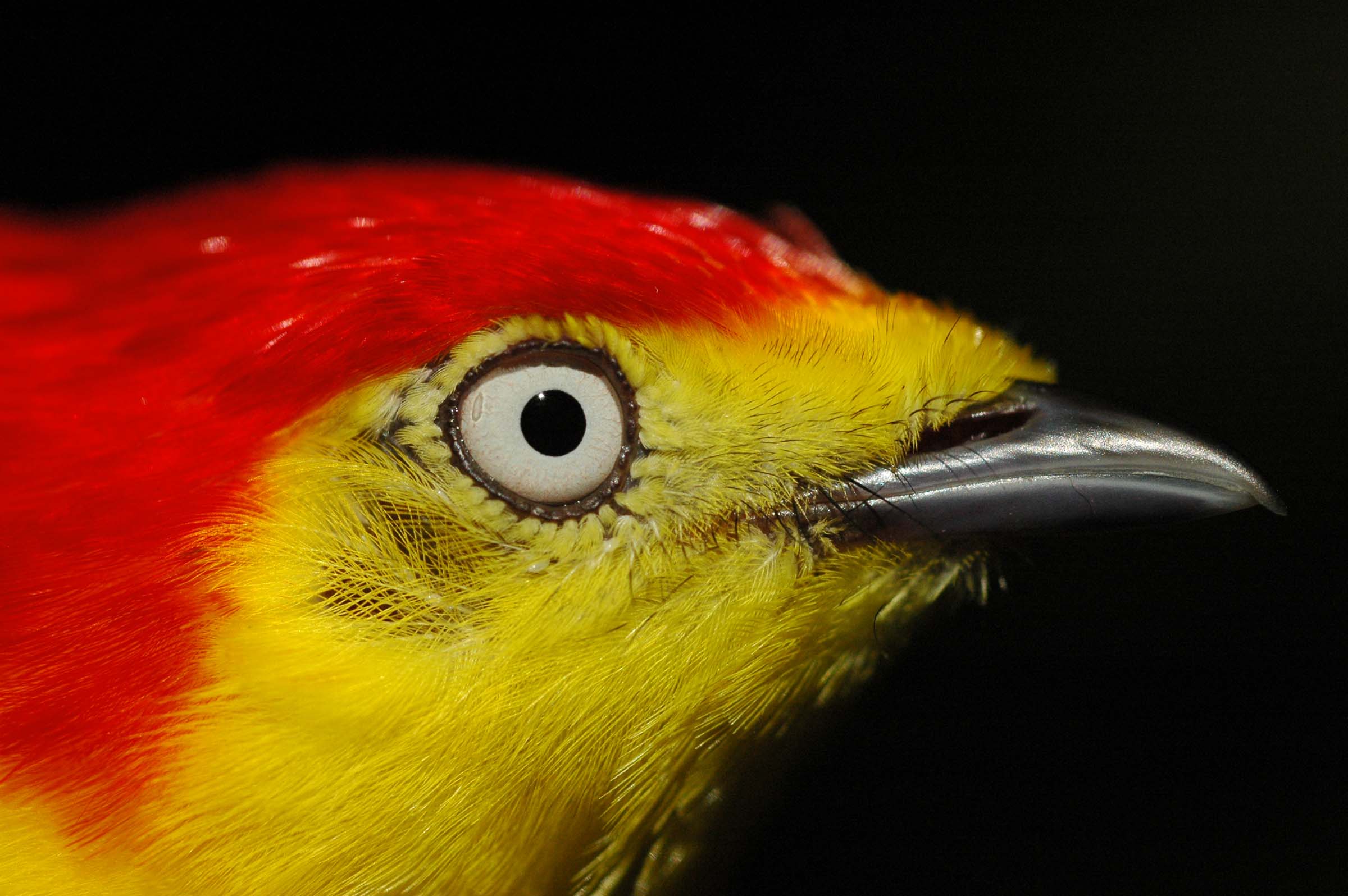The image is a highly detailed, close-up portrait of a bird's head against a solid black background. The bird is positioned in profile, looking to the right. Its vibrant feathers are meticulously rendered, whether in a photograph or in hyper-realistic art. The upper portion of the bird's head is adorned with vivid red feathers, reminiscent of bright cherry or fruit punch red, which sweep backward in a striking crest. Directly beneath the red, the feathers transition to a brilliant yellow that extends around the eye and covers the lower part of the head and chest. 

The bird's eye is a focal point, reflecting light and surrounded by a series of colored rings: a black pupil, encircled by white, and then brown. The beak is a glossy black, with light reflecting off both the upper and lower parts, making it appear almost silver due to its shine. Fine whisker-like feathers extend towards the beak, adding to the intricate detail. The overall composition, highlighted by the stark black background, accentuates the bird's striking coloration and detailed features, suggesting it could be of tropical origin.